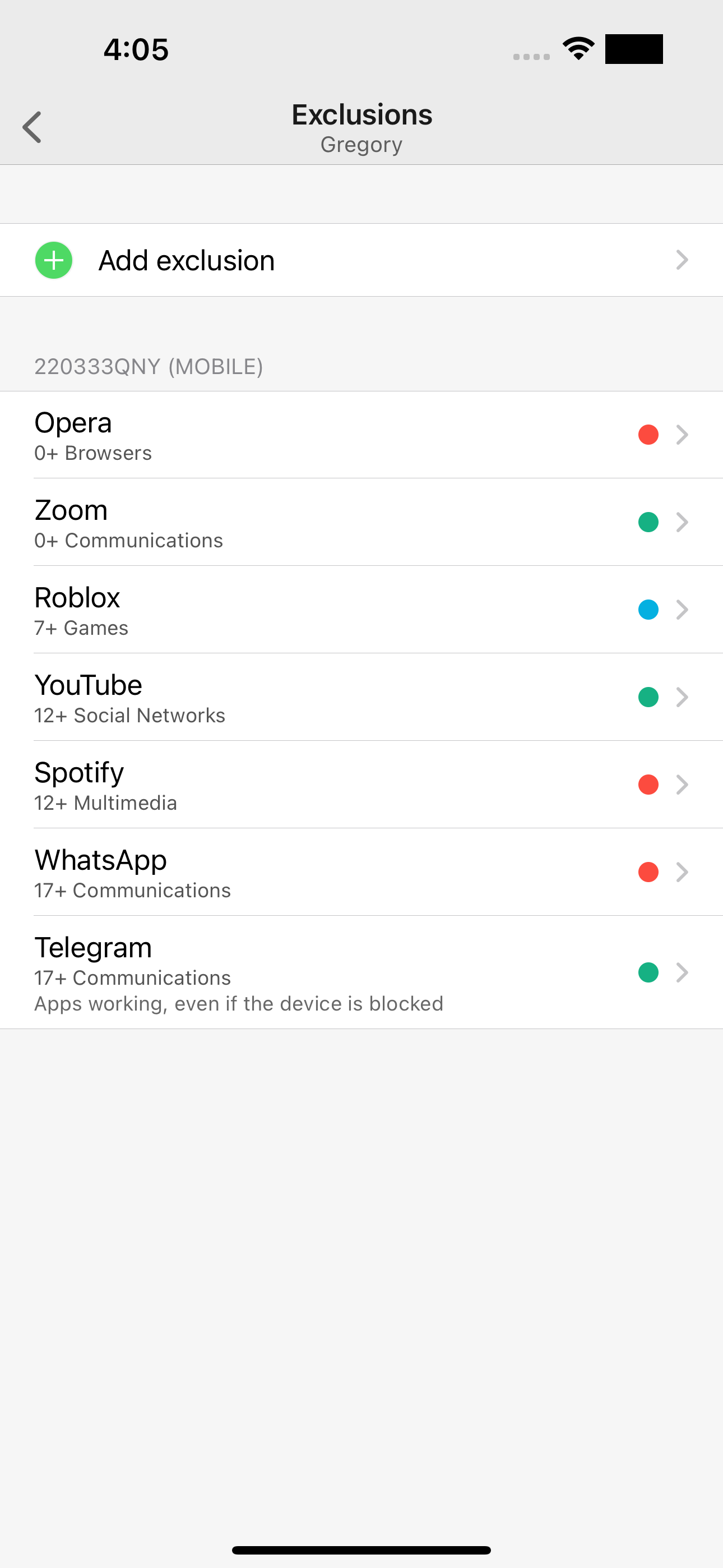The screenshot depicts various interface elements on a mobile phone. In the top left corner, the time is displayed as "4:05". Directly opposite, in the top right corner, there are four grey dots representing something and a Wi-Fi signal icon. Below this, a horizontal black box is present.

Underneath this, on the left side, a left-pointing arrow icon is visible. Centrally aligned, bold black text reads "Exclusions," with "Gregory" written below it in dark grey. Beneath this, there's a white bar; on its left is a green circle with a white plus sign, followed by the text "Add Exclusion" in black. At the bar's right end, a grey arrow points to the right.

Following this, a grey area contains the text "22033QNY" with "(Mobile)" beside it in black. Below this, "Opera" is written in bold black, followed by "0 + Browsers" to the right. A red circle with an arrow pointing to the right accompanies the text.

Next, several items are listed, each featuring a colored circle with an arrow:

1. "Zoom" followed by "0 + Communications" to the right with a green circle.
2. "Roblox" followed by "7 + Games" to the right with a blue circle.
3. "YouTube" followed by "12 + Social Networks" to the right with a green circle.
4. "Spotify" followed by "12 + Multimedia" to the right with a red circle.
5. "WhatsApp" followed by "17 + Communications" to the right with a red circle.
6. "Telegram" followed by "17 + Communications" and "Apps working, even if the device is blocked" to the right with a green circle.

At the bottom center of the page, a black horizontal line approximately three inches long is positioned.